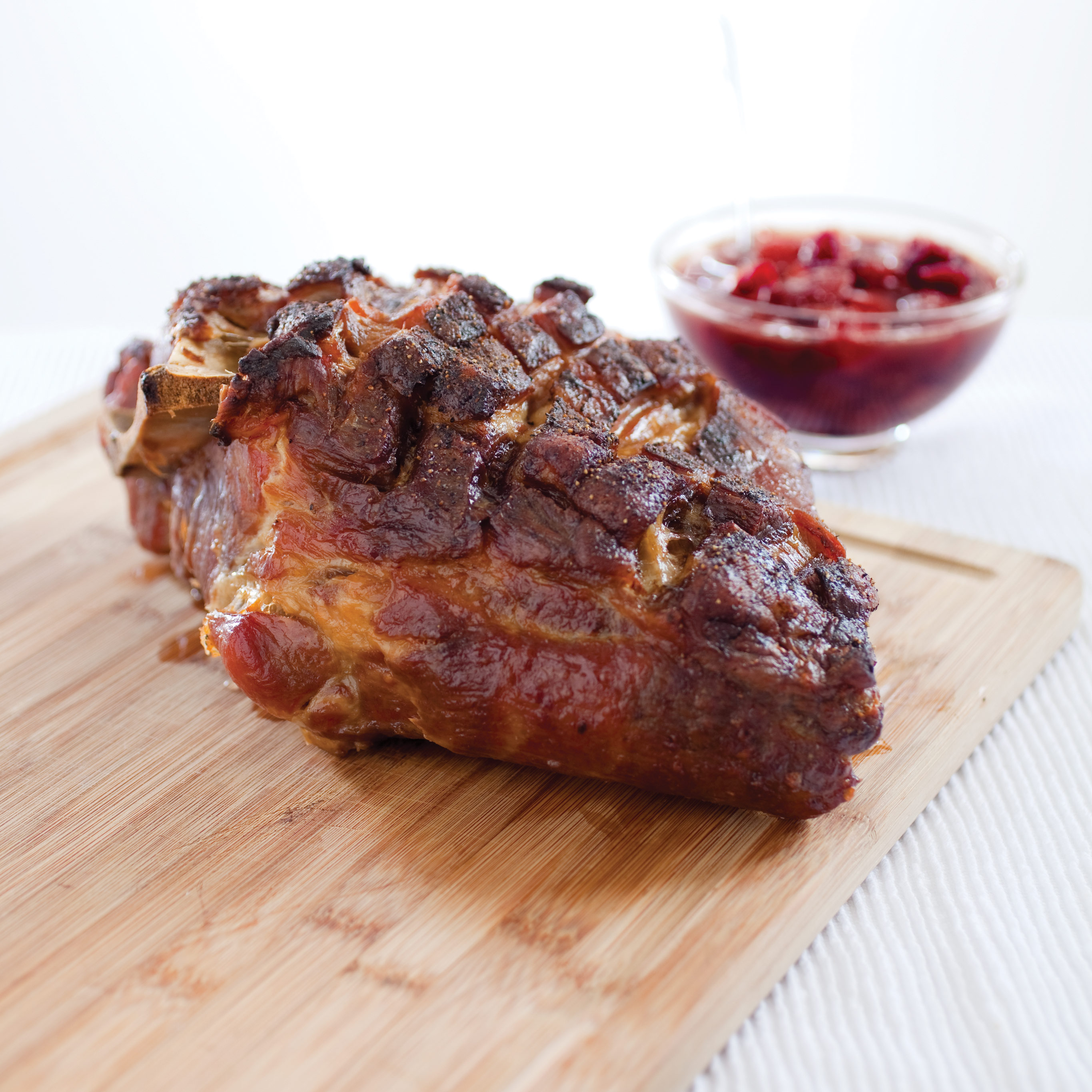The image features a cooked piece of meat, possibly a pork roast or ham, characterized by its thick, glazed surface with detailed texture and a reddish-brown color. The meat rests on a wooden cutting board, which sits atop a non-stick mat on a white surface, potentially a tablecloth. The meat has hints of slightly cooked fat, some brown bits, and areas with whitish-yellow coloration, possibly indicating bone or cartilage. In the blurred background, there is a clear glass bowl containing a reddish liquid and chunks of red fruit, adding depth to the otherwise focused image of the succulent meat.